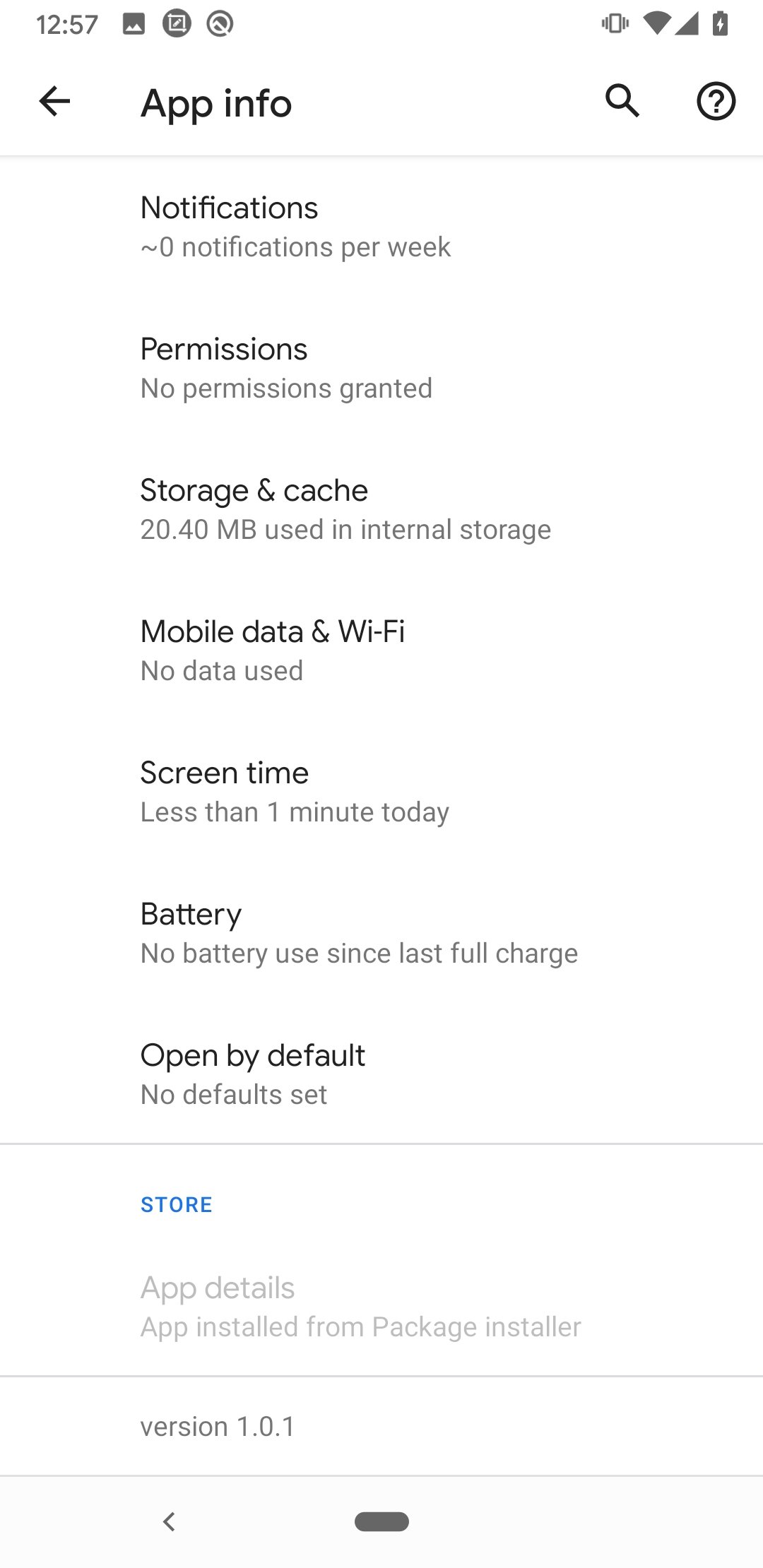This image captures the screen of an unspecified device with a predominantly white background. At the top left corner, the time is displayed as 12:57. Adjacent to it on the right are four icons, arranged from left to right: a vibrate icon, a wireless icon, a cellular signal icon, and a battery icon. 

Below this, on the left side of the screen, there is a black arrow pointing to the left, accompanied by the text "App Info." On the right side at the same level, two more icons are visible: a magnifying glass and a question mark. 

Further down, the screen displays the following details in a structured manner:

- **Notifications**: "Notifications: 0 notifications per week"
- **Permissions**: "No permissions granted"
- **Storage and Cache**: "0.40 MB used in internal storage"
- **Mobile Data and Wi-Fi**: "No data used"

This detailed layout provides an overview of the application's current status and settings.